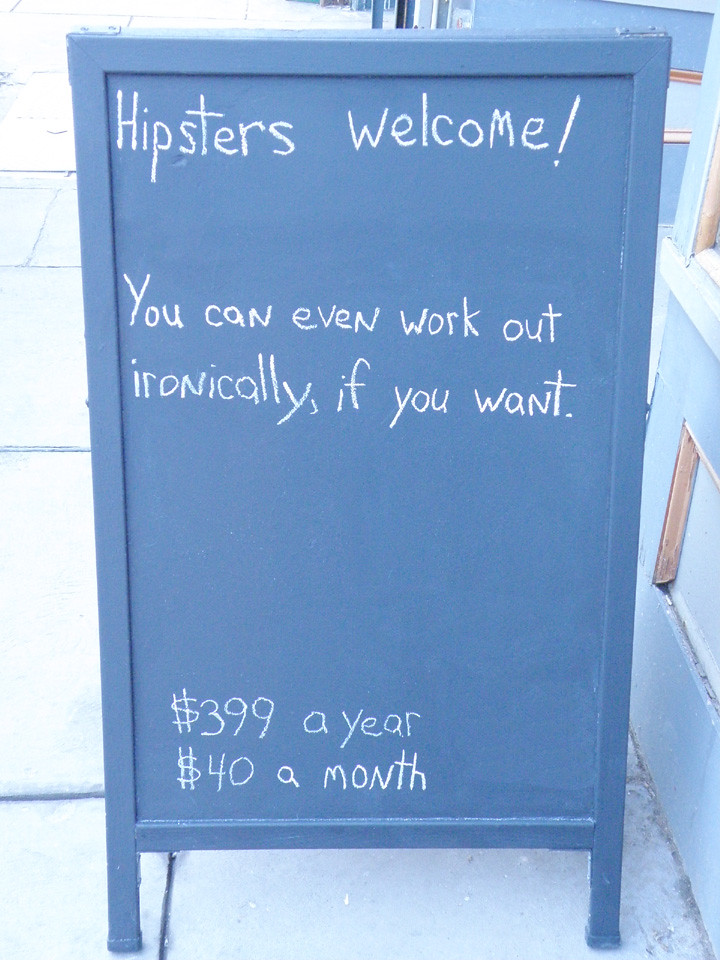This blue poster board sign, likely an advertisement for a gym, is situated outside on a sidewalk, adjacent to a building with a light blue wall and white trim to the right. The sign, standing on two short legs, features a simple design with all text handwritten in white chalk. At the top, it boldly proclaims "HIPSTERS WELCOME!" with an exclamation mark. Further down, in the middle of the board, it humorously notes, "You can even work out ironically, if you want," spread across two lines. The bottom of the sign provides membership details: "$399 a year," with "$40 a month" noted directly underneath. The scene appears washed out due to extreme daylight, making the white text stand out prominently against the dark charcoal gray or blue background of the poster board.